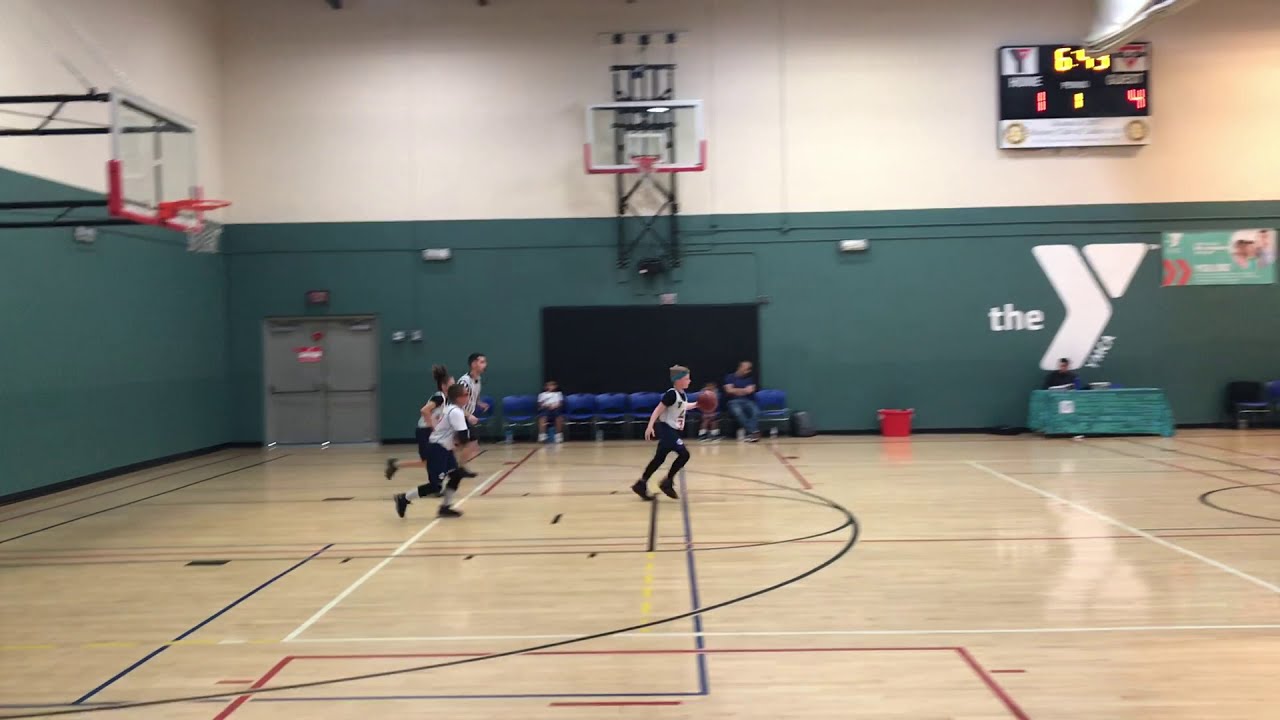The photograph captures an indoor basketball game at a YMCA gymnasium. The gym's lower walls are green while the upper half is white, prominently displaying the word "THE" followed by a stylized letter "Y," shaped like a right-facing arrow and an upside-down triangle, with "YMCA" inscribed on the right side of the Y. The light wooden basketball court is marked with red, white, and blue lines. Four young children are running towards the right, dressed in white jerseys and black pants. The back wall features a row of blue seats where three spectators are sitting, including a young child in shorts and a white t-shirt, and an adult in darker attire. On the right side, near a green table, a man dressed in black is seated. The entire setting is brightly lit, providing a clear view of the scene despite minor blurring in some parts. The gym also includes basketball hoops, emergency exit doors, and various indoor lights illuminating the activity.